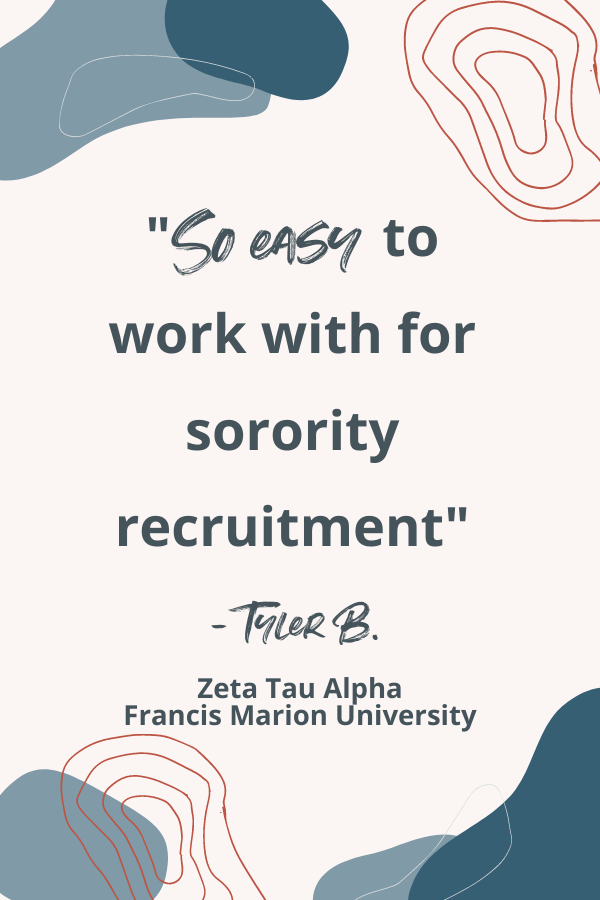The image showcases a glowing testimonial highlighting its ease of use for sorority recruitment, quoted as: "So easy to work with for sorority recruitment." The quote is attributed to Tyler B., with the affiliation details "Zeta Tau Alpha, Francis Marion University" displayed beneath it in blue letters against a light cream background. The text features a script-type font with a paintbrush stroke design, primarily in black or dark blue.

The background is adorned with various abstract shapes and patterns: red squiggly lines forming nested ovals in the upper right, wavy navy blue and light blue blobs on the left, and more red lines paired with dark blue waves in the lower-left and right corners respectively. These elements contribute to the visually engaging and artistic composition, enhancing the overall aesthetic appeal of the testimonial.